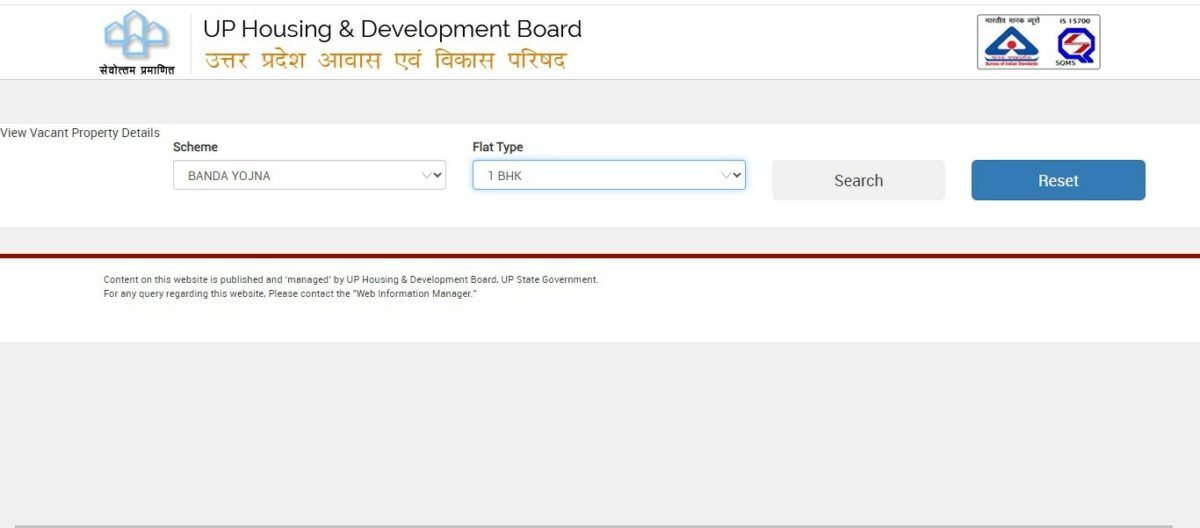This is a detailed screenshot of a specific website interface. At the top, there's a prominent white navigation bar stretching across the full width of the screen. On the left side of this bar, there is a logo composed of a group of four homes outlined in light blue, with accompanying text in a foreign language, possibly Arabic. Adjacent to the logo, additional text in Arabic script is present. Toward the right side of the white bar, two visually distinctive badges are located: one features a blue triangle with a red dot, while the other resembles a speech bubble with a red lightning bolt inside it.

Beneath this section, there is a gray horizontal bar. Directly below this, the section labeled "Vacant Property Details" begins. Within this section, two drop-down menus are available: one labeled "In Scheme" with the option "Bandayuchna," and another labeled "Flat Type" with the option "1BHK." Next to these drop-down menus is a gray "Search" button and a blue "Reset" button.

(Note: The closing phrases appear to pertain to a video sign-off that is unrelated to the context of the screenshot and have been omitted from the descriptive caption for clarity.)